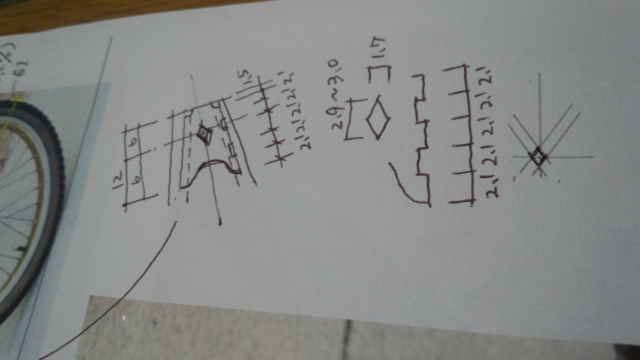This photograph features a white background adorned with intricate pen drawings and mathematical notations. On the right side, several numbers, such as 2.1 and 1.7, are rotated counterclockwise, suggesting that the image or the numbers may be oriented sideways. 

The left side of the image prominently displays a detailed drawing of half a bicycle wheel. The wheel is depicted with a black outer tube, contrasting with the white inner section. Golden spokes fan out from the center, adding a touch of realism to the sketch. Below the wheel, a curved black line arcs downward from the bottom left towards the center, roughly bisecting the lower portion of the image.

There appear to be diagrams and diverse shapes scattered across the page, along with additional numbers like 12, 6, and 19 situated in various locations. A black dividing line runs horizontally beneath the bicycle tire, contributing to the composition's structured yet chaotic aesthetic. The bottom part of the image hints at a marble countertop texture, adding an intriguing element to the illustration. The overall atmosphere of the photograph is slightly dark, enhancing the contrast and depth of the drawings.